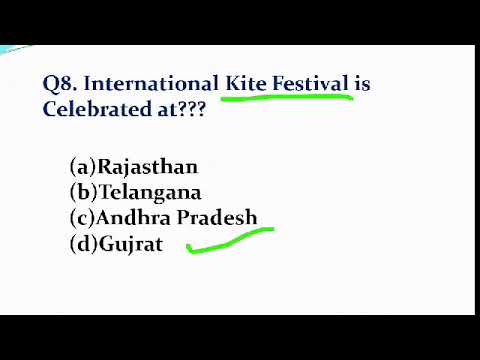The image is a computer screen displaying a slide with a white background and thin black borders on the top, bottom, and right sides. In the top left corner, there's a small blue triangular mark. Centered on the page, in dark blue or black text, it reads, "Q8 International Kite Festival," with "Kite Festival" underlined in green. Below this, it says, "was celebrated at ???" The text is followed by a list of four multiple-choice options:

A. Rajasthan (R-A-J-A-S-T-H-A-N)
B. Telangana (T-E-L-A-N-G-A-N-A)
C. Andhra Pradesh (A-N-D-H-R-A P-R-A-D-E-S-H)
D. Gujarat (G-U-J-R-A-T), which has a green check mark beside it.